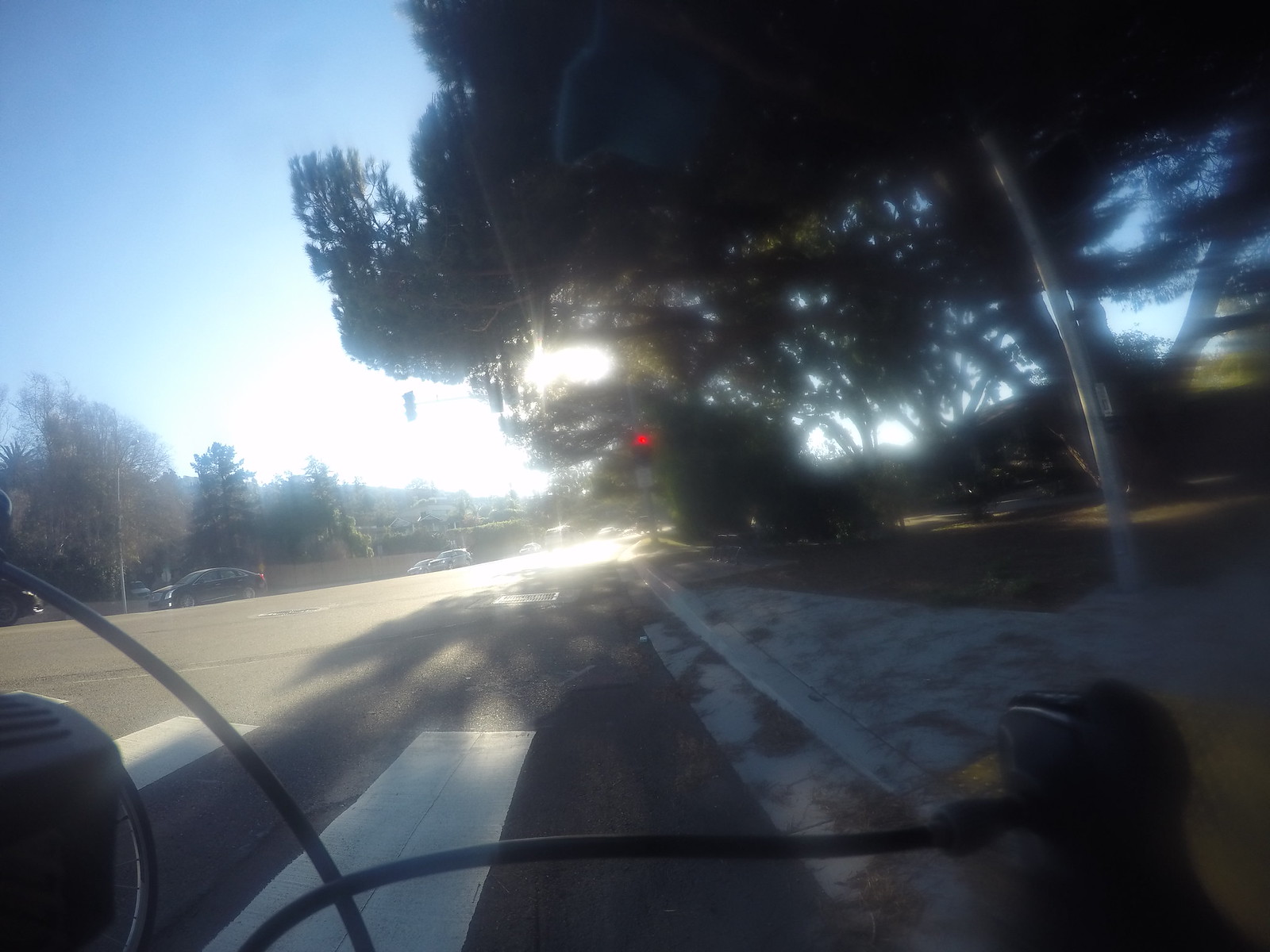The image is a blurry daytime photograph, seemingly taken from the perspective of someone seated on a motorcycle on the right-hand side of a lane. Directly in front of the viewer, there are black and white pedestrian crossing lines. The photograph shows a red traffic light up ahead, with cars visible in the distance heading diagonally to the left. To the right of the lane, there is a sidewalk bordered by bushes and trees, with sunlight filtering through the foliage. A streetlight, silver in color, is also visible near the trees. In the foreground, hoses are connected to something sitting on a black shape on the curb. The sky is light blue, suggesting the sun may be setting behind the trees in the center background. The trees on both sides dominate the view, appearing mostly dark due to the lighting, with just a hint of colors from the leaves and sunlight.